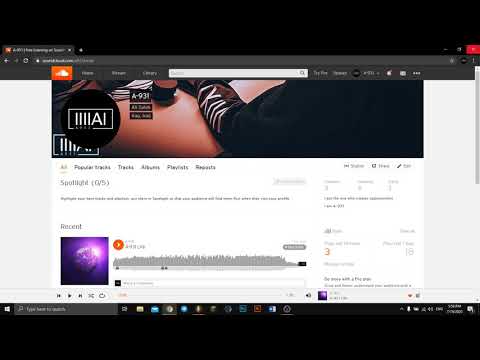The image depicts a zoomed-in view of a SoundCloud webpage open in a web browser. Despite the blurriness, you can distinguish the key elements of the interface. At the top, SoundCloud's recognizable rectangular orange icon with the white cloud is visible. To the right of the icon, there are three black bars indicating a menu, followed by a search bar and several clickable elements. 

Below this header, the content on the screen features a dark object with white stripes, possibly a person's arm, and a black oval logo. Within this black oval, there is a white rectangle containing four vertical white lines on its left side, a prominent capital letter "A," and a vertical line. Under this section, there is a clickable play button intended for video playback.

Though pixelated due to the zoom, the SoundCloud branding and interface layout are evident.